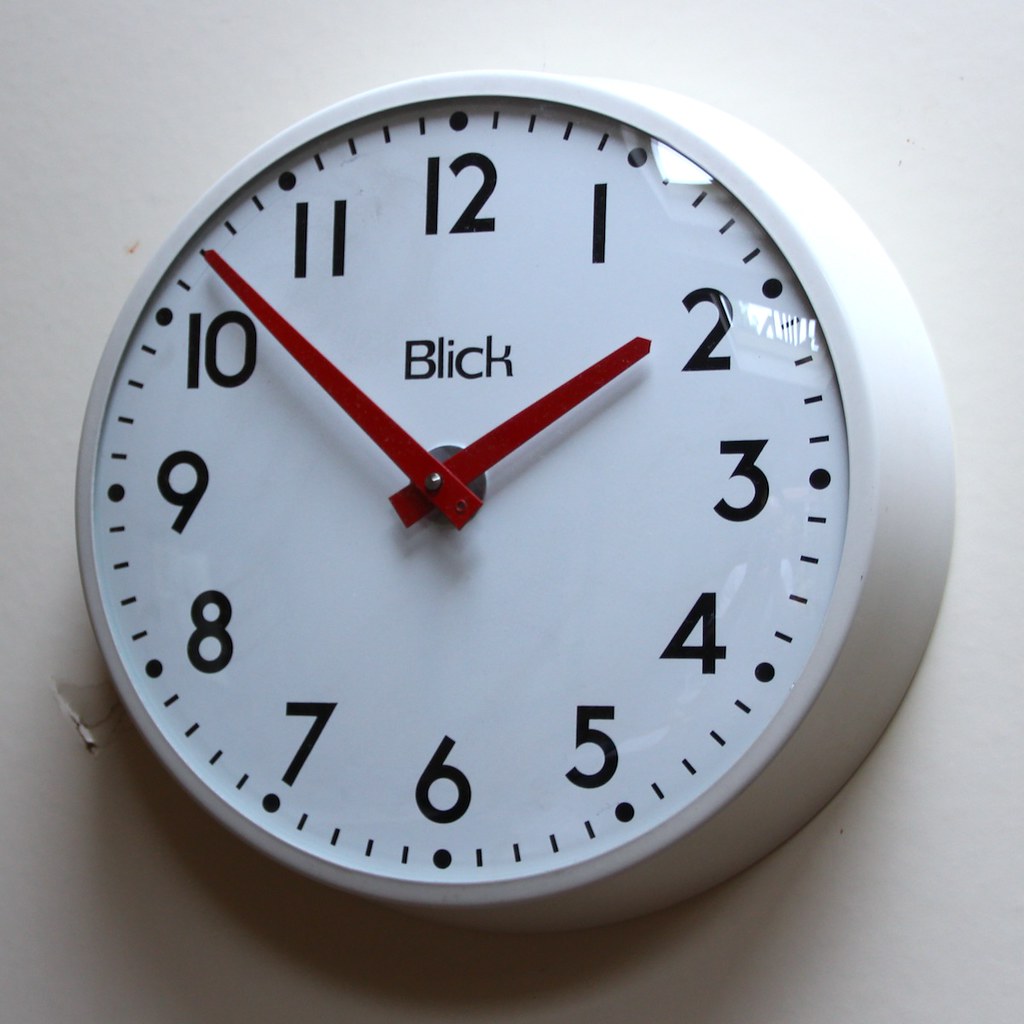This detailed image shows a round wall clock made by the company Blick, with the brand name "Blick" clearly visible between the center of the hands and the 12. The clock features a white face with black numerals, and each minute is marked—those on the hours with black circles and the rest with narrow lines. The hour and minute hands are both bright red, narrowing and angling to a point at the tip. Currently, the time reads 1:52, or eight minutes until 2 o’clock.

The clock is encased in a white plastic or metal frame that slightly angles out towards the wall it hangs on. The face is protected by a glass or clear plastic cover, which reflects light and possibly windows from the surrounding environment, especially noticeable near the one and two o’clock markers.

The clock is mounted on a plain white wall that shows evident signs of wear. Notably, there is a hole or a chip near the left side of the clock, around the 8 o'clock position, as if someone bashed it with a hammer. Additionally, the wall has some paint peeling and dirty elements. A shadow from the clock is cast below due to the lighting coming from the upper right corner, enhancing the overall stark and somewhat worn appearance of the scene.